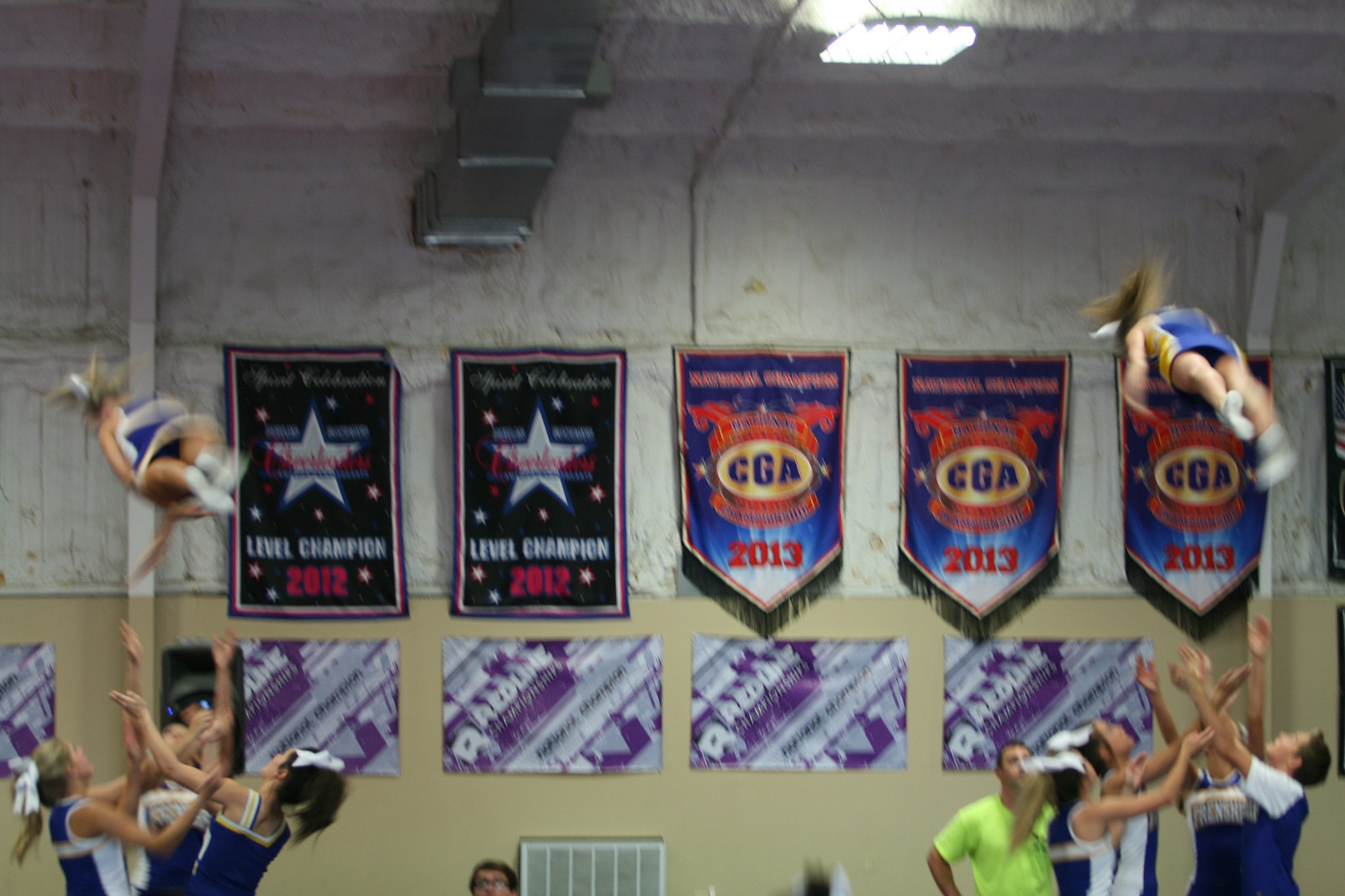The photograph captures an energetic scene inside a gymnasium used for cheerleading practice. The gym's upper walls are cement gray, transitioning to a beige color on the lower half, adorned with a series of banners. Notably, the wall features white and purple rectangular banners inscribed with "Red Line," and above them are several championship banners, including black rectangular banners with white stars that proclaim "Level Champion 2012," as well as pointed-bottom banners labeled "CGA 2013."

Flanking either side of the image are two groups of cheerleaders donned in blue, white, and yellow uniforms with white bows in their hair. Each squad is dynamically tossing a flyer into the air. The group on the right includes a man, possibly a coach, wearing a bright yellow T-shirt with his hands on his hips, attentively watching the performance. In the background and around the edges of the gym, a few spectators can be seen. The bright overhead lights illuminate the vigorous practice session, highlighting the precision and coordination of the cheerleaders in mid-action.